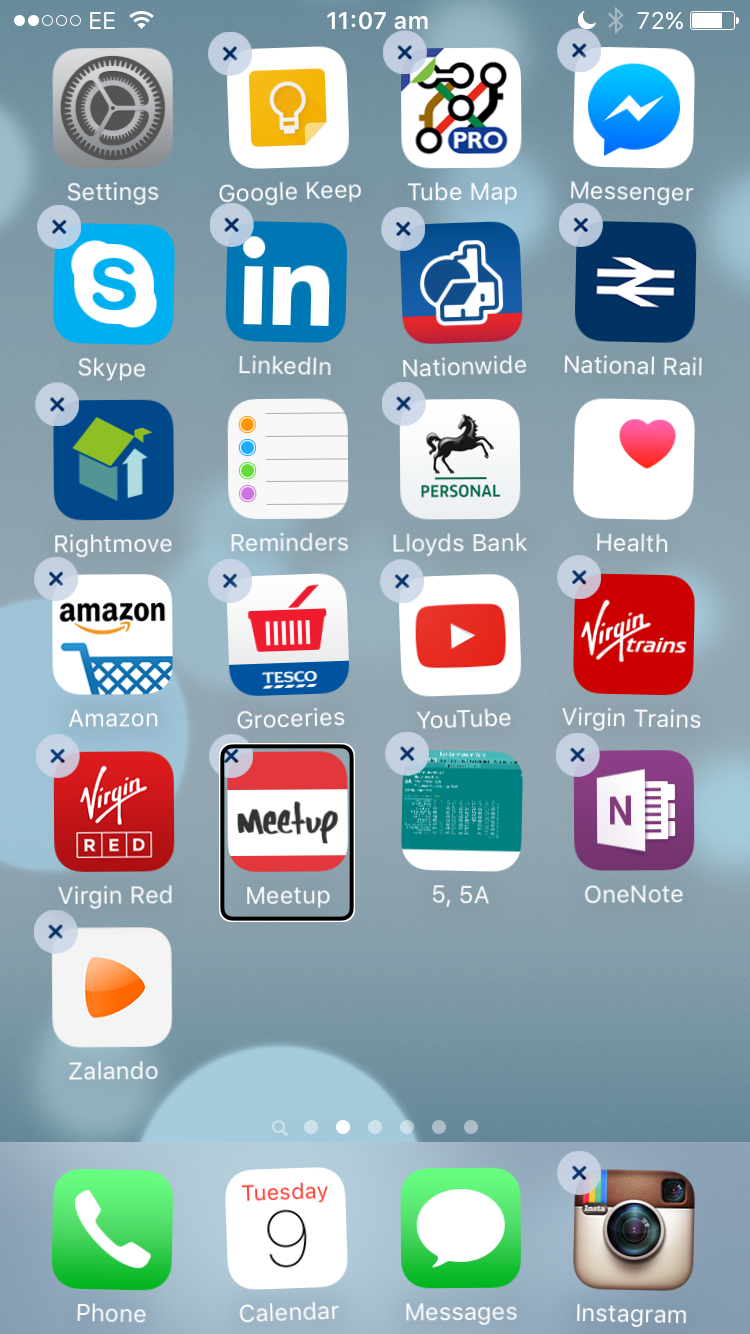The image showcases an iPhone home screen with a distinctive, aesthetically pleasing background. The top of the screen displays the time "1707 AM" in white text. The overall theme is a serene, pale blue-gray, adorned with varying sizes of translucent circles that resemble bubbles. These bubbles have a subtle gradient effect, transitioning from a very light, pale blue to a slightly darker, teal-ish blue.

At the bottom of the home screen, within a gray rectangular dock, the user has placed their primary apps: the Phone app, Calendar app, Messages app, and Instagram app, arranged from left to right in their standard iPhone icon appearances.

Above the dock, there is a search icon flanked by a series of white dots, each representing a different page of apps. This specific home screen contains a total of 25 app icons, neatly organized and contributing to the clean, minimalistic look of the user's interface.